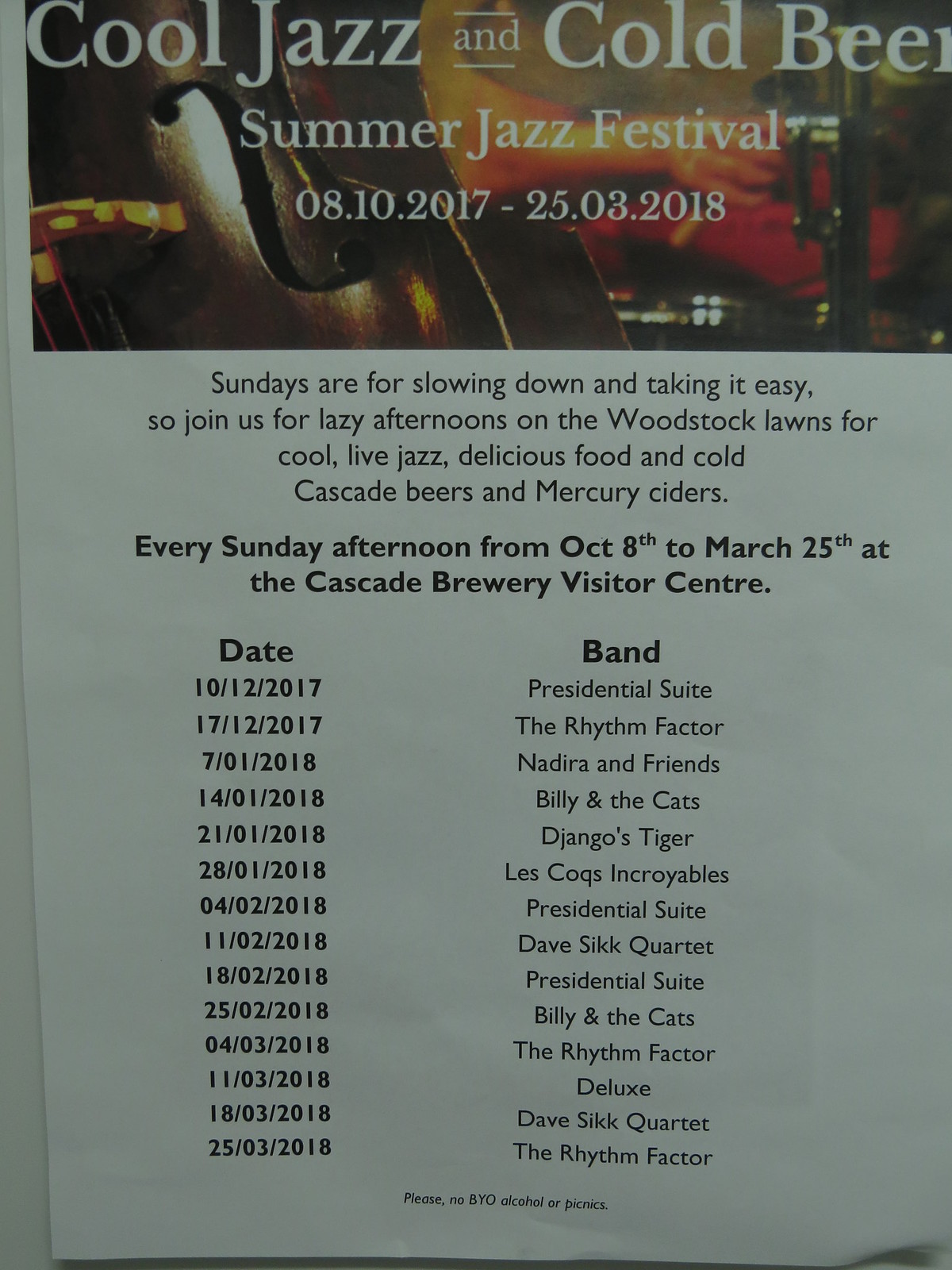This advertisement showcases the "Cool Jazz and Cold Beer Summer Jazz Festival," prominently displaying the headline in white ink against a backdrop featuring a violin and wind instruments. The event details span from August 10, 2017, to March 25, 2018, with the festival promoting a relaxed atmosphere perfect for lazy Sunday afternoons on the Woodstock Lawns. Visitors are invited to enjoy live jazz performances, delicious food, and cold Cascade beers and Mercury ciders every Sunday from October 8th to March 25th at the Cascade Brewery Visitor Center. A detailed list of performing bands is included, featuring names such as Presidential Suite, The Rhythm Factory, Nadir and Friends, Billy and the Cats, among others. The advertisement concludes with a note advising that no BYO alcohol or picnics are allowed.